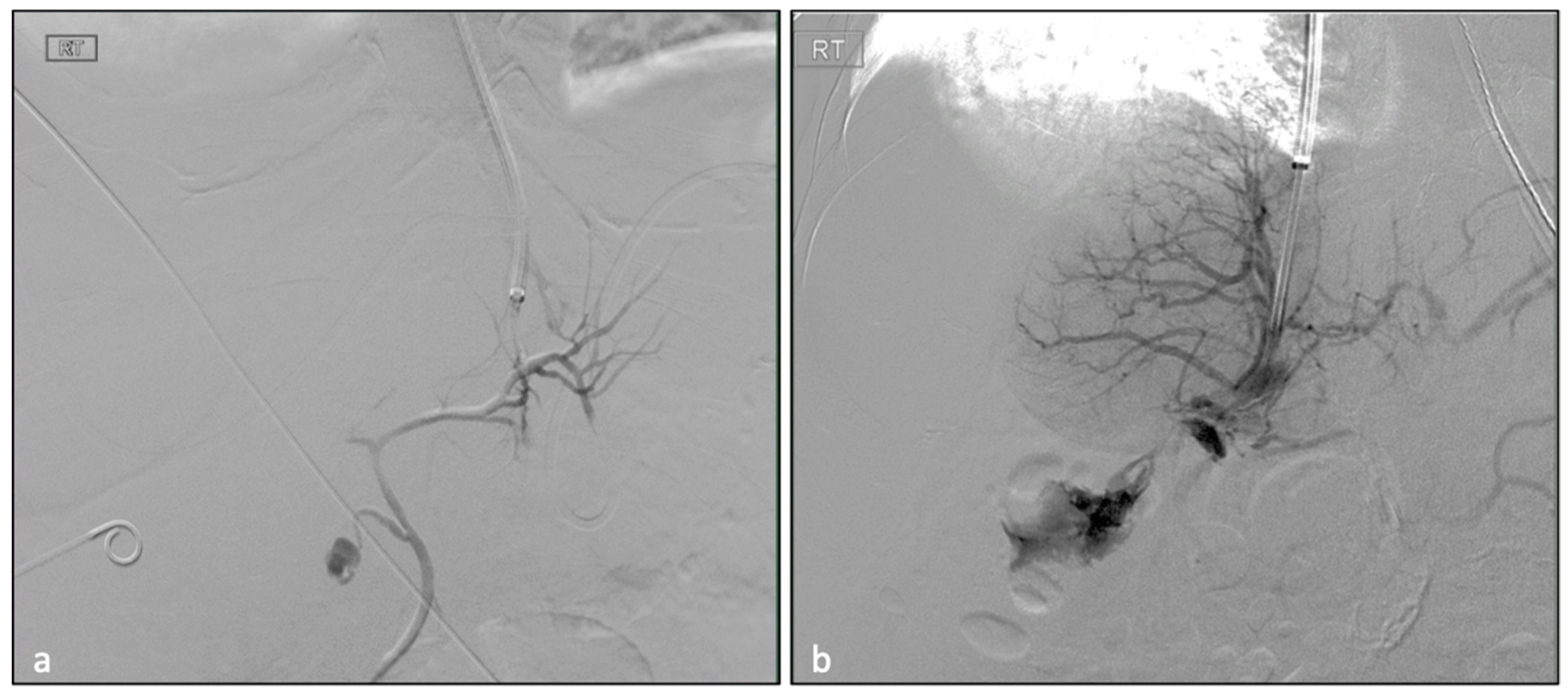The image consists of two side-by-side grayscale photographs, each labeled with white lettering - "A" and "B" - and "RT," which likely stands for real-time. The left photograph (A) depicts a detailed, curving structure resembling a tree or root system. This structure starts from the bottom, arches left and right, and then branches out extensively, resembling arteries or veins captured through some form of imaging, possibly an x-ray or microscopic imaging. The right photograph (B) shows a similar background and an equally intricate, tree-like network. This network extends from top to bottom, resembling a tube feeding into the branching system. Both images share a complex, organic appearance, with dark tree-like patterns contrasted against a lighter gray background, suggesting either biological veins, capillaries, or possibly even bacterial growth captured in high detail.